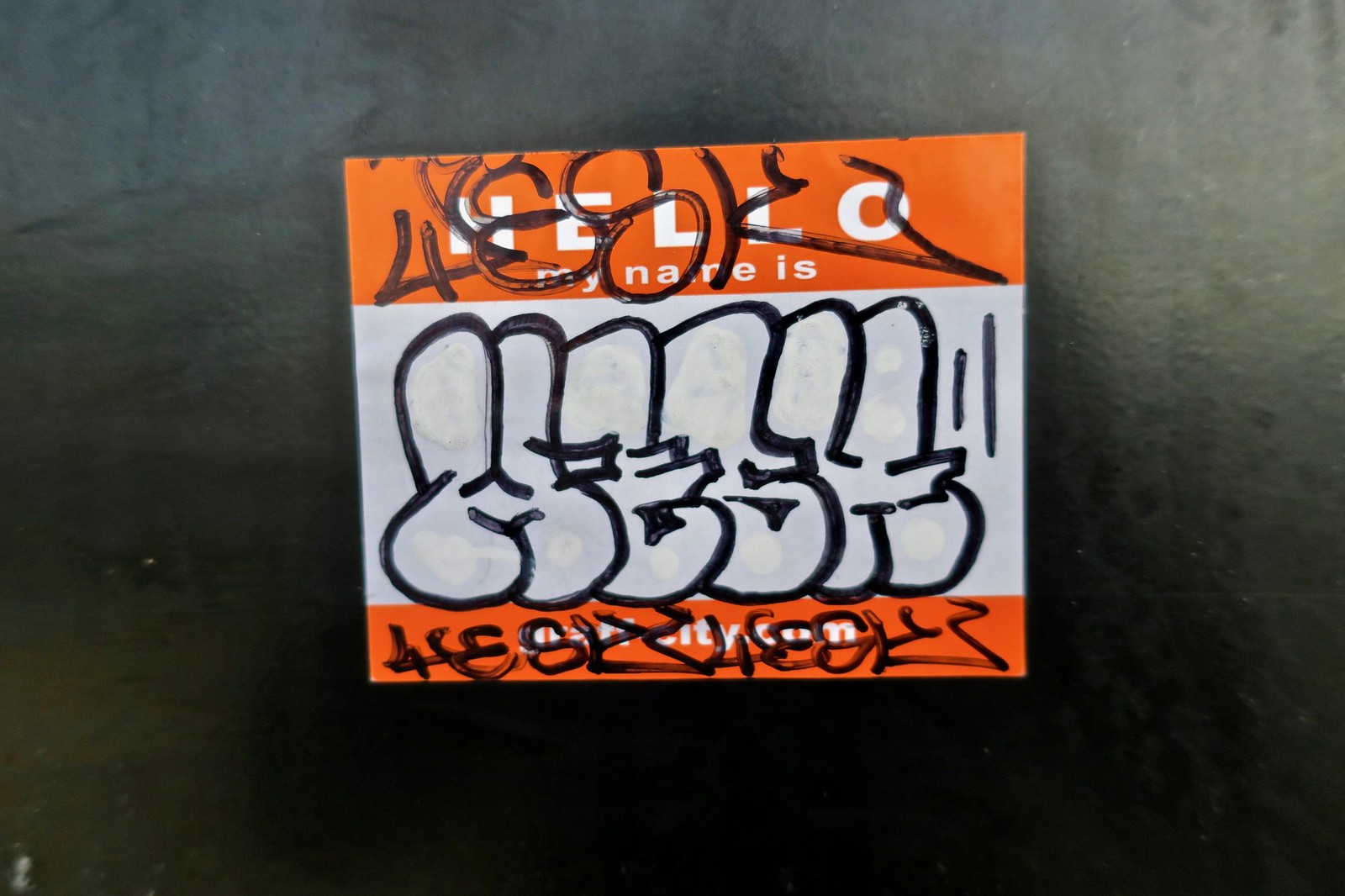This close-up image features a "Hello, my name is" name tag sticker typically worn at conventions or meet-and-greets. The sticker is placed against a black surface, which could be a table or a wall—the close proximity of the shot leaves this detail ambiguous. The top of the sticker has an orange band with the printed text "Hello, my name is," while the bottom orange band includes the text "city.com." The first part of the bottom text is mostly obscured by ink, but fragments like "G-R-A" and possibly "F-T" are visible. The central white space of the sticker, meant for writing a name, is defaced with various graffiti markings made with a Sharpie. This graffiti includes what appears to be alphanumeric characters such as "488K," and other illegible sketches or symbols that might depict a series of figures pointing to the right. The words and images in the center are against a lighter background but are largely indecipherable, possibly written in another language or non-standard script, resembling comic sans font. The vandalism on the sticker amalgamates random letters and abstract drawings, creating a chaotic and hard-to-interpret scene.